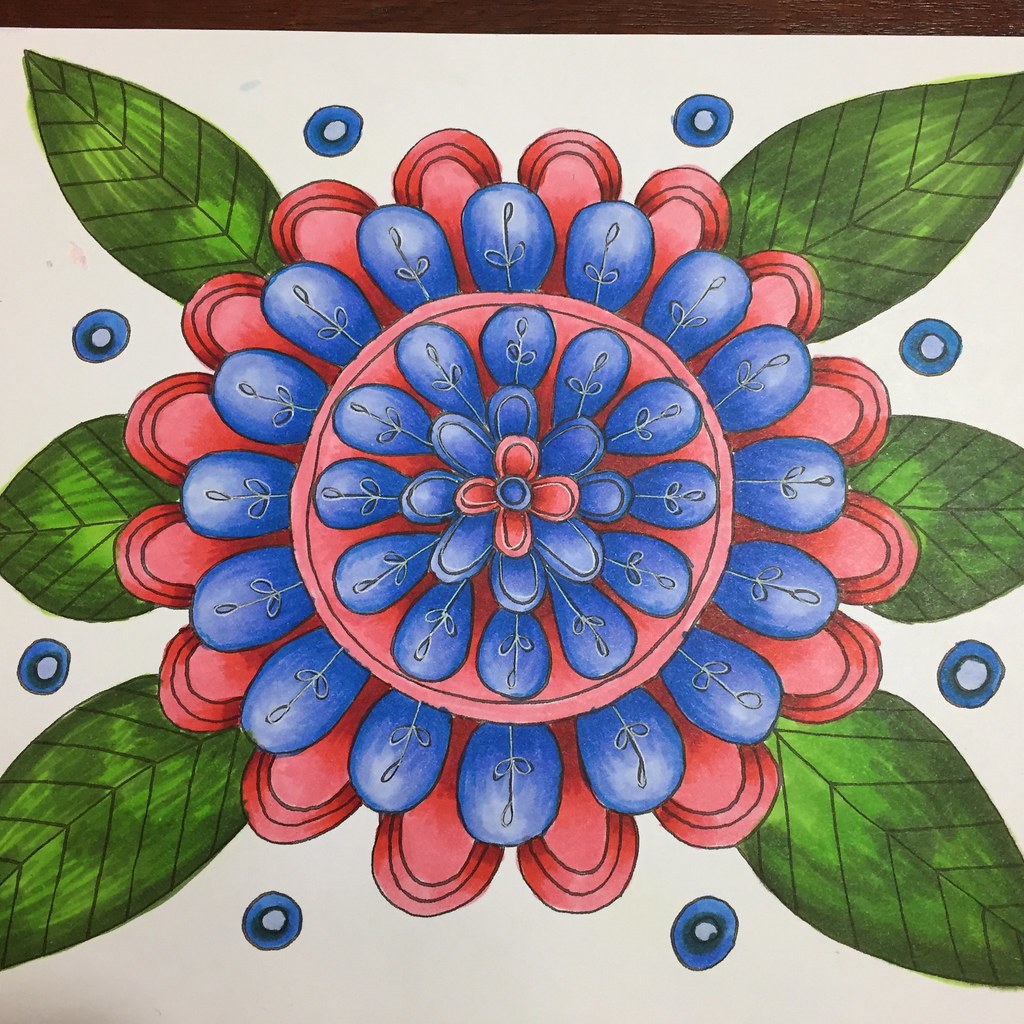This intricate drawing showcases a plant meticulously illustrated on white paper. The plant features six verdant leaves, symmetrically arranged with three on each side. Each leaf is detailed with a central vein and a pattern reminiscent of elongated V shapes. Interspersed throughout the illustration are eight circles, each a vibrant blue with a central white hole, adding a dynamic element to the piece.

Connecting the leaves to the plant's core are flowers adorned in shades of pink and red, adding depth and a splash of contrasting color. Progressing towards the plant’s center, blue petals emerge, each intricately decorated with a delicate white design. This pattern repeats, leading to a layer of blue petals devoid of any white detailing, enhancing the complexity of the arrangement.

At the very heart of the plant lies a striking red bloom, its small leaves extending outward in cardinal directions. The central focal point of the composition is marked by another blue circle, anchoring the entire artwork with a sense of completeness and balance.